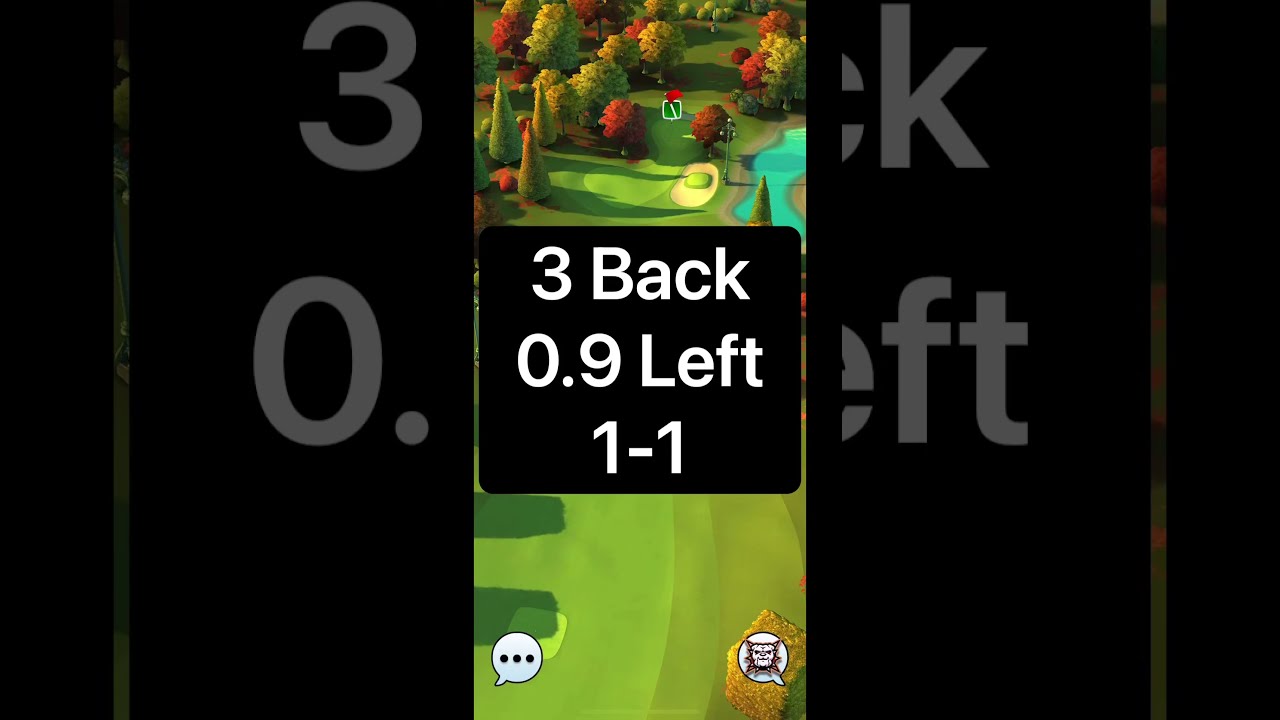This vertically oriented, narrow rectangle image appears to be a screenshot from a mobile video game, possibly a golf game. The top section of the image showcases a detailed and colorful golf course, featuring trees in varying shades of green to red, a water pond, a putting green, and a house or cottage structure positioned centrally. Midway through the image, there is a prominent black square box with white text displaying: "3 back," "0.9 left," and "1-1." The lower third of the rectangle appears to be the driving green or tee area, where the player would initiate their shot. In the bottom left corner, there is a chat bubble with a white background and three black dots inside. The bottom right corner features a white circle containing a cartoon-style lion, which likely serves as the player's avatar.